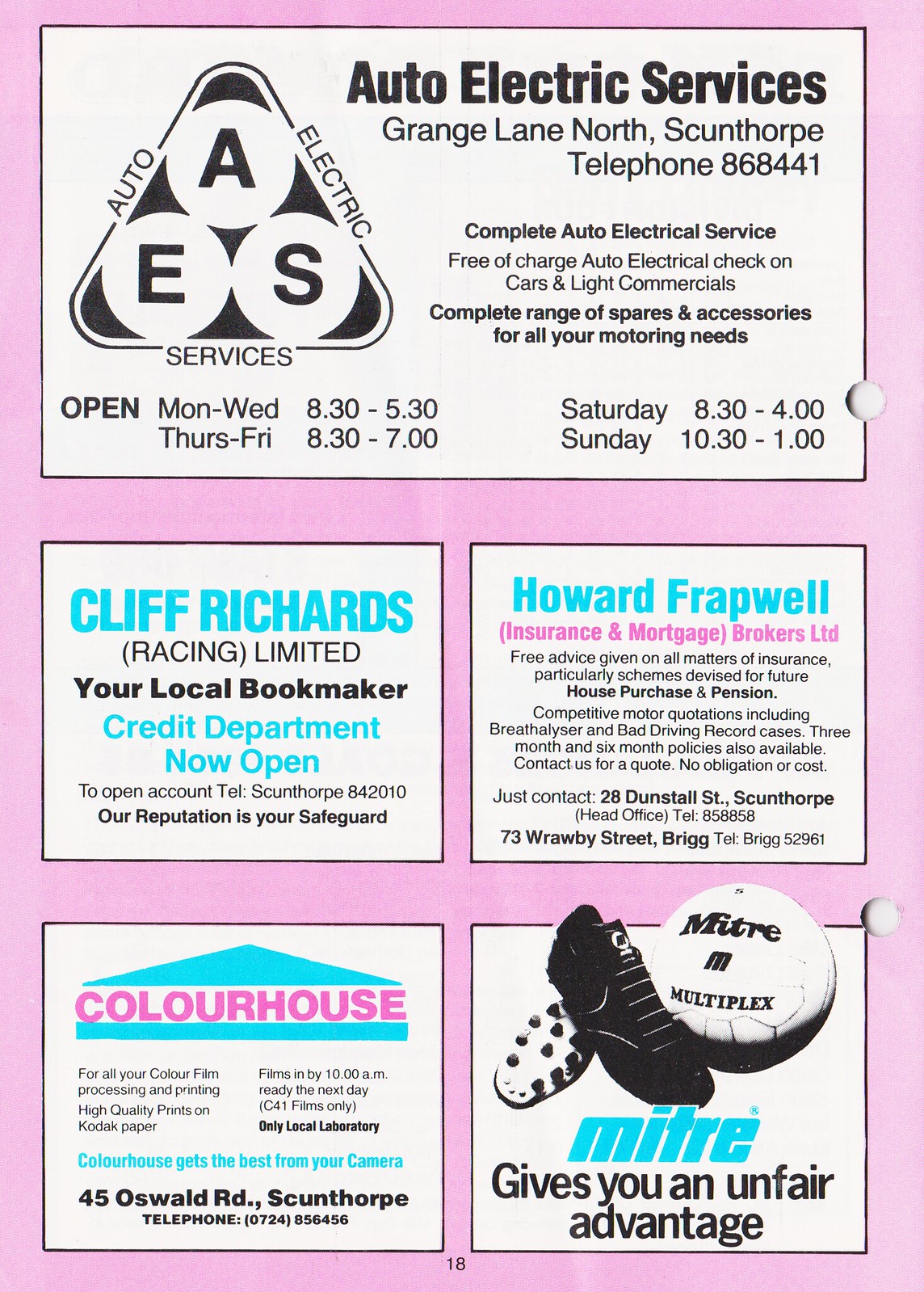The image appears to be a pink page from a phone book or magazine, indicated by a page number "18" at the bottom center. At the top, it features a prominent advertisement for "Auto Electric Services," located at Grange Lane North, Scunthorpe, with telephone number 868441. The business card-like ad includes their logo, a triangle with the letters AES (each within a white circle), stacked and arranged to form a stylized frame. The ad details their comprehensive auto electrical services, including free checks for cars and light commercials, a full range of spares, and accessories. Their operating hours are Monday to Wednesday from 8:30 AM to 5:30 PM, Thursday to Friday from 8:30 AM to 7:00 PM, Saturday from 8:30 AM to 4:00 PM, and Sunday from 10:30 AM to 1:00 PM.

Below this, the middle section contains two side-by-side advertisements. The left ad is for "Cliff Richards Racing Limited," described as the local bookmaker, now offering services through their credit department, accompanied by their contact information and slogan. The right ad is for "Howard Frapwell Insurance and Mortgage Brokers Limited," featuring a couple of paragraphs elaborating on their services.

The bottom section has two more advertisements. The left ad is for "Color House," which specializes in color film processing and printing, displayed within a blue house-shaped logo and accompanied by an address. The right ad, titled "MITRE," promotes sports equipment with the tagline "Mitre gives you an unfair advantage."